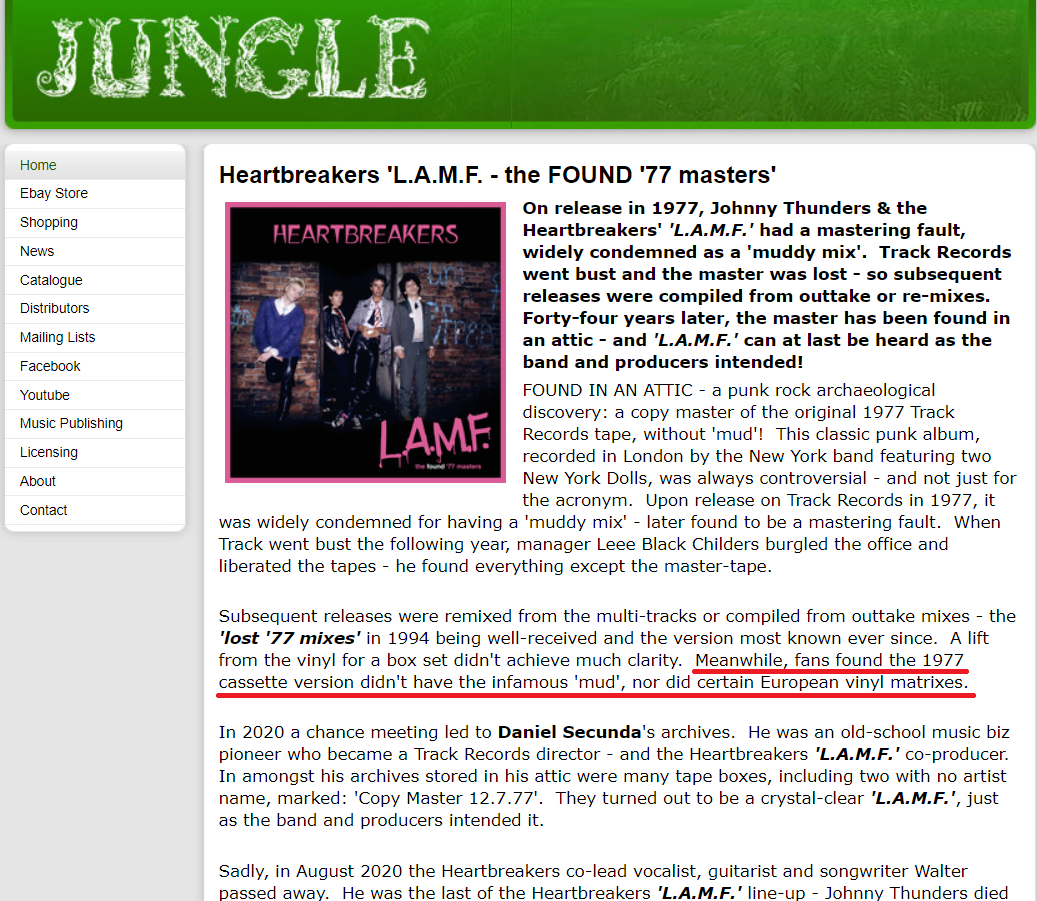Screenshot of an older version of a web page featuring a green navigation bar across the top with the word "Jungle" displayed in white and green letters. On the left side of the navigation bar, there is a menu with links in green and black text including "Home," followed by a list of options: eBay Store, Shopping, News, Catalog, Distributors, Mailing Lists, Facebook, YouTube, Music Publishing, Licensing, About, and Contact.

The main content of the page is a detailed article titled "Heartbreakers L.A.M.F - The Found '77 Masters," which discusses a musical band. Most of the text is in black, with some bolded for emphasis. A notable line is underlined in red, stating "Meanwhile fans found the 1977 cassette version didn't have the infamous mud nor did certain European vinyl matrices."

Embedded within the article is an image, presumably the front cover of an album. The cover is outlined in pink and features four people standing against a wall. The title "Heartbreakers" is prominent, with "L.A.M.F" noted in the bottom right-hand corner of the album cover.